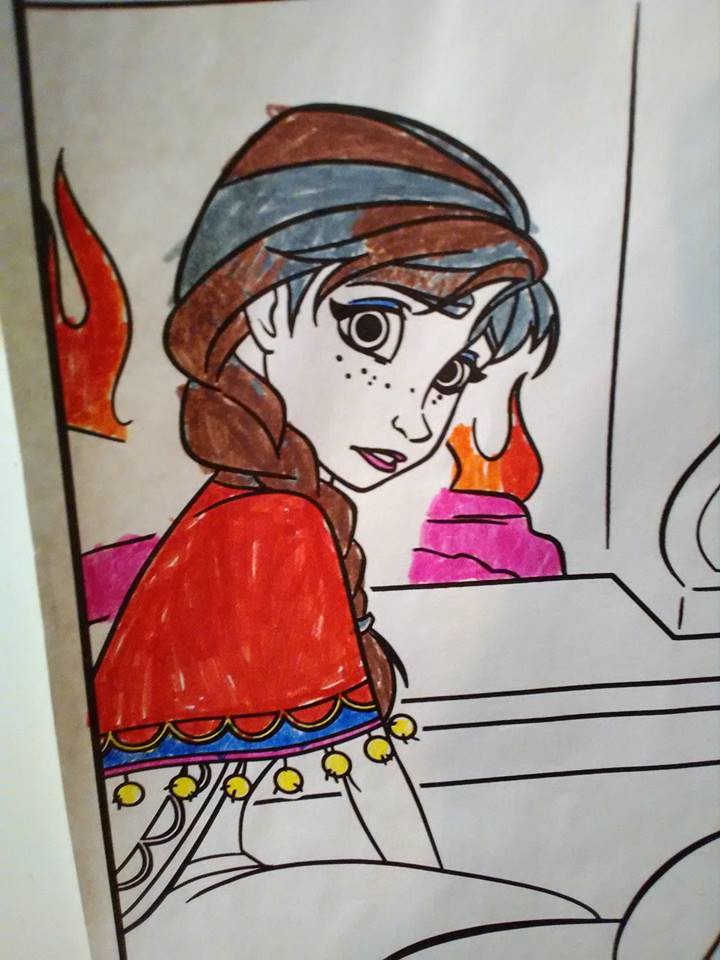This image appears to be a page from a children's coloring book, featuring a character with a Disney princess-like appearance, possibly Anna from Frozen. The character is colored with distinctive brown and gray hair, adorned with blue eyeshadow and freckles. She wears a red shawl draped over her shoulders, which is detailed with yellow tassels. The background features an image of orange flames, adding warmth and contrast to the black and white line work that remains uncolored.